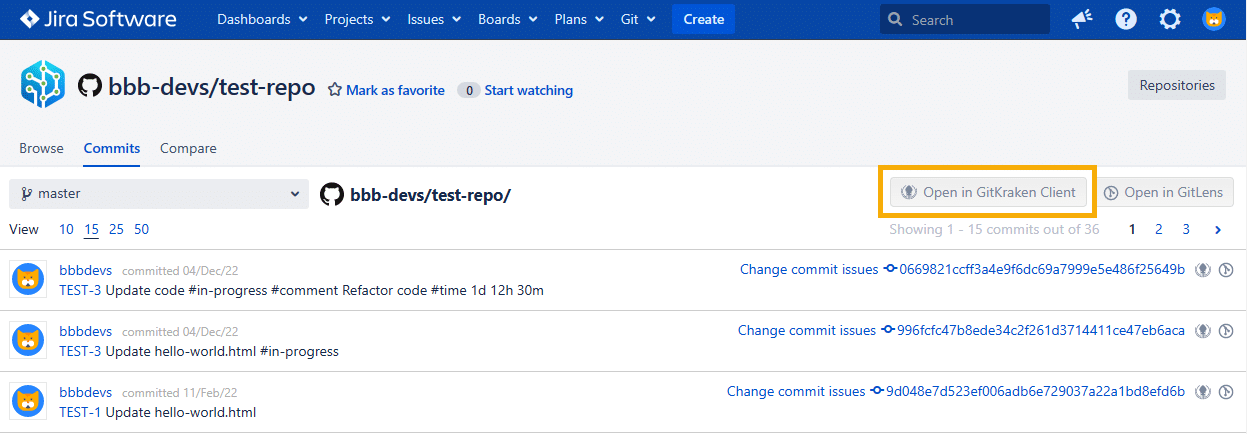This image is a horizontally oriented screenshot displaying the interface of a software company’s application, specifically Jira Software. At the top of the image is a dark blue banner that prominently reads "Jira Software," accompanied by a diamond icon to the left. To the right, the banner features several drop-down categories labeled "Dashboards," "Projects," "Issues," "Boards," "Plans," and "Git," along with a "Create" button and a search bar. 

In the top right-hand corner, there are four icons or logos. Below the banner, the main header section has a light gray background and is titled "BBB/devs/test-repo." Additionally, there are options to "Mark as Favorite" and "Start Watching." Adjacent to these options, on the right side of the column, is a gray button labeled "Repositories."

The "Commits" category is selected, displaying a vertical column with three listed tests under "BBB devs." Each test entry is depicted inside a horizontal box with an icon of a cat in a blue circle, followed by clickable blue links. The content is spread over pages two and three. The overall color scheme of the interface includes white, light gray, and various shades of blue, providing a clean and professional look.